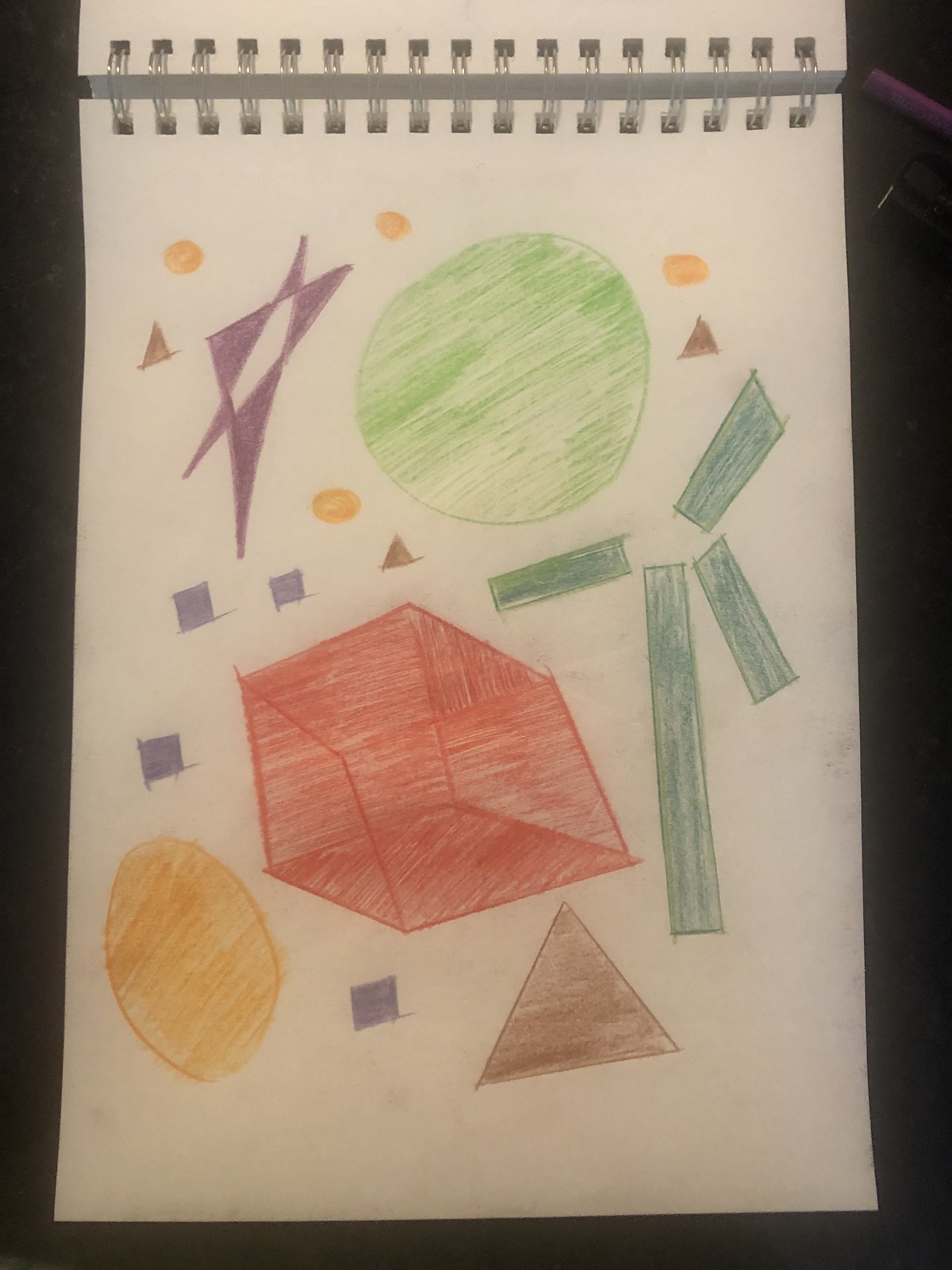The caption you provided has been cleaned up and elaborated into a detailed descriptive caption:

---

A delightful page from a child's sketchbook, placed vertically against a black background, showcases an array of colorful shapes drawn with colored pencils. The sketchbook's spiral rings are prominently featured at the top of the page. From the top going across, the artwork begins with two small golden-orange circles. Directly beneath them is a vibrant purple star, accompanied by a brownish triangle. To the right, a light green circle adds a refreshing touch of color. Continuing the pattern, another orange oval appears, juxtaposed with another brown triangle. Moving further down, four elongated blue rectangles are arranged in sections. Below them, an awkwardly shaped red cube stands out. To the left of the cube, there are blue-violet squares, and below these squares, a golden oval shines brightly. The composition concludes with additional blue-violet squares and a larger brown triangle. This playful collection of shapes captures the joyful creativity of a child's imagination.